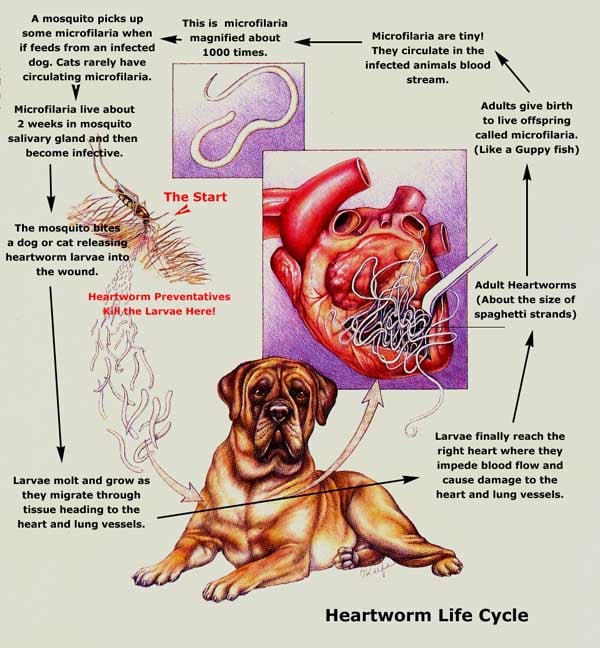This is a detailed vertical infographic poster about the heartworm life cycle, typically found in a veterinarian's office to educate dog owners. The top of the poster features an enlarged image of a heartworm, which is long and white, almost resembling a tangled ball of yarn. The primary section of the poster graphically illustrates a dog's heart, interlaced with heartworms, depicted in a vivid red with yellow highlights and a purplish border, emphasizing the severe impact of the infestation.

In the foreground stands a large, tan-colored dog, which appears to be suffering from heartworm, framed against a light green background. Surrounding this central image are paragraphs of text and arrows that guide the viewer through the stages of the heartworm life cycle in a circular pattern. It begins with a mosquito picking up microfilariae from an infected dog and continues through the various developmental phases within the mosquito before transferring the larvae into another dog or cat.

Infographic details explain that microfilariae live for about two weeks in a mosquito’s salivary gland before becoming infective. Once transferred to a new host, the larvae migrate through tissue toward the heart and lung vessels, growing and molting, as depicted in intermediate images around the dog's heart. Below the dog image, the caption explicitly states "heartworm life cycle," highlighting the lengthy and twisted journey of the heartworm in graphic, informative detail.